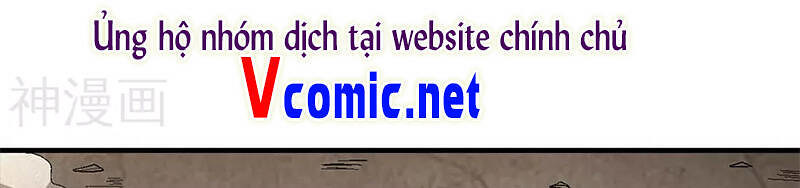The image is a long, horizontal, rectangular banner that seems designed for a website. It has a predominantly white background with centered text. The text is in an Asian language, likely Vietnamese, reading "UNG HO NHOM DICH TAI website CHINH CHU," with some characters featuring accent marks and dots. Below this text, in the left section of the image, there's a prominent red capital "V," followed by "comic.net" in a cold blue color. Additionally, there are various Asian characters to the left of this text. The bottom part consists of a black stripe adorned with small drawings—such as lines and flat triangles—that span over a brown-gray area, resembling the ground or a wall with subtle designs and patterns.